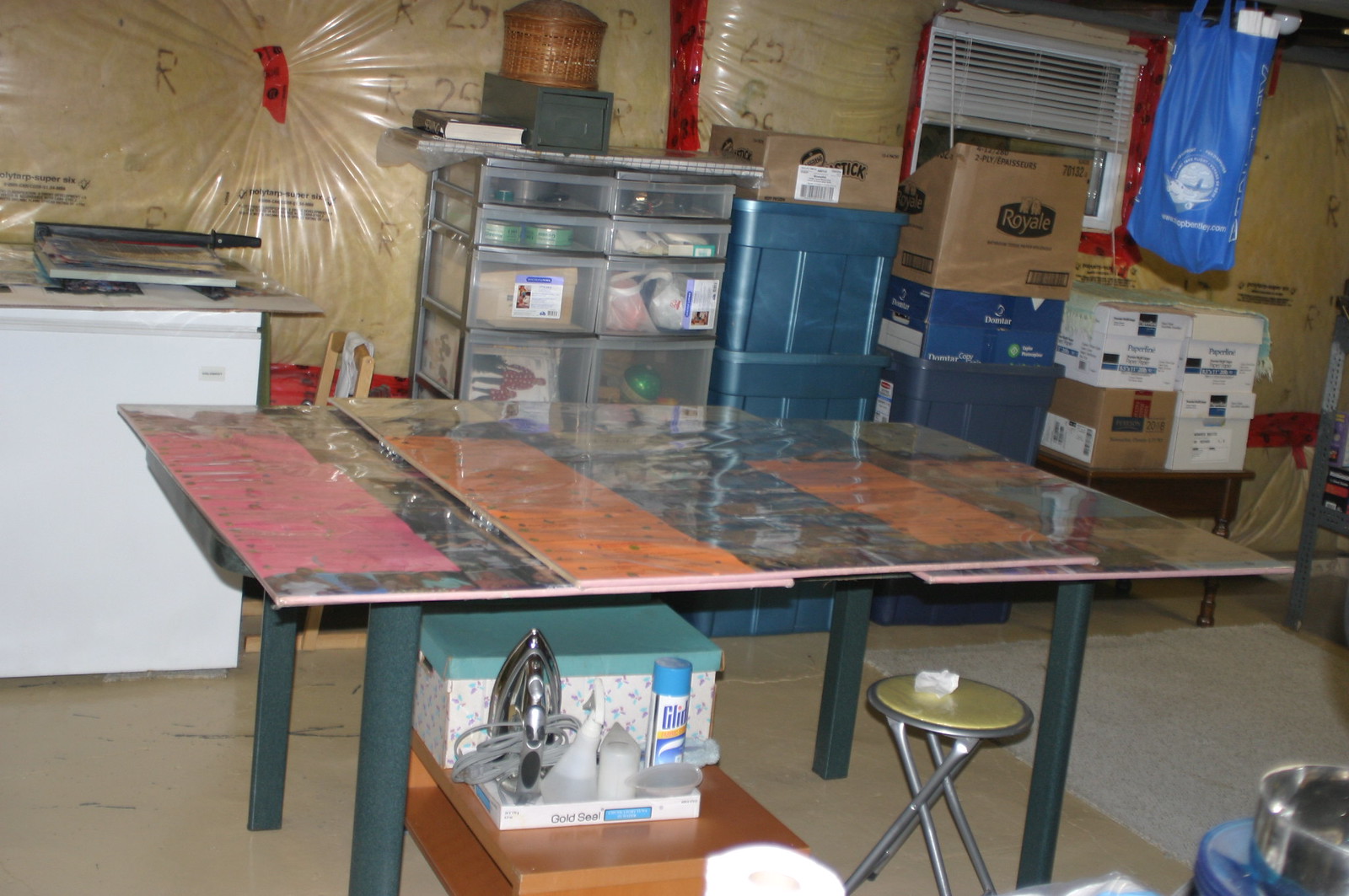In this dimly lit photograph taken indoors, the setting appears to be a storage room or possibly a stock room of a business, likely snapped at night given the dark, open window with open blinds in the upper right corner. The focal point of the image is a large table situated in the center of the room, completely covered by a poster board adorned with various images, although the exact details are indiscernible due to the angle. Underneath the table, various items are visible including several boxes, cans of dust spray or a similar product, an iron, and a small stool. 

The background reveals meticulously organized storage, featuring numerous neatly stacked plastic Rubbermaid-style totes, plastic organizers, and additional boxes. The room’s walls appear unfinished, draped in plastic wrap revealing brown paper beneath it. Hanging from the ceiling in the upper right, there is a blue and white bag, adding to the eclectic assortment of the stored items. The overall ambiance of the room is that of a well-used, yet meticulously organized storage space, bathed in a dim, nocturnal glow.